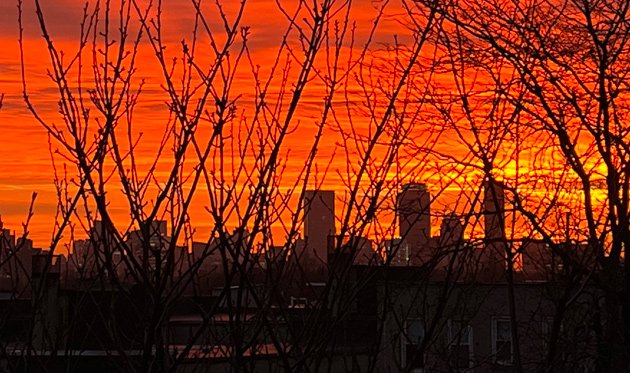The image captures an expansive urban skyline, potentially of New York City, dominated by an array of buildings stretching from the foreground to the distance. Prominent tall buildings, including what appears to be the post-9/11 structure, stand out, indicating a sizable metropolis. The top 60% of the picture showcases a cloudy sky, suffused with the brilliant hues of an orange and yellow sunrise or sunset, casting a warm, glowing light across the scene. This vibrant glow creates an ethereal backdrop, with horizontal cloud formations adding to the dramatic effect. Branches from leafless trees in the foreground partially obstruct the view, suggesting it is either fall or winter. These branches, though plentiful, are not dense enough to conceal the intricate details of the cityscape. In the mix, various power lines add to the urban complexity, juxtaposed against the natural beauty of the brilliant sunrise/sunset. Overall, the photograph is a stunning blend of architectural marvels and natural splendor, framed by the skeletal silhouettes of barren branches.